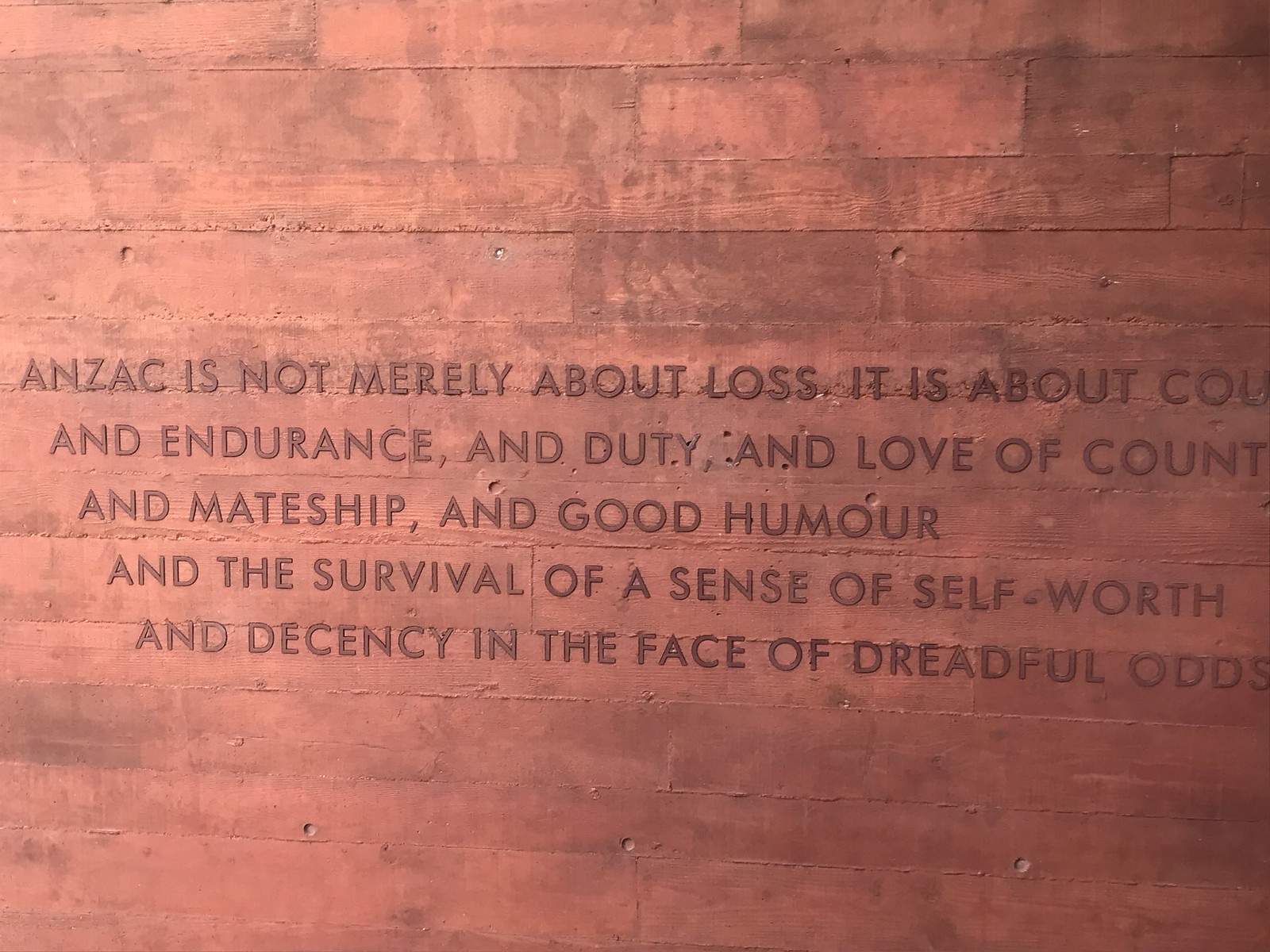The photograph depicts a wall with a brick-colored background, though it might be wooden slats painted to resemble brick. The wall has small regular holes, adding to its textured appearance. Centrally affixed to the wall is an inscription composed of five lines of text, in dark brown or darker red letters that stand out clearly against the background. The text is written in all capital letters in a simple English font, and reads:

"Anzac is not merely about loss, it is about courage and endurance, and duty, and love of country, and mateship, and good humor, and the survival of a sense of self-worth and decency in the face of dreadful odds."

The inscription emphasizes concepts like endurance, duty, love, mateship, good humor, and maintaining self-worth and decency despite challenging circumstances. There are no other images or faces present in the picture.